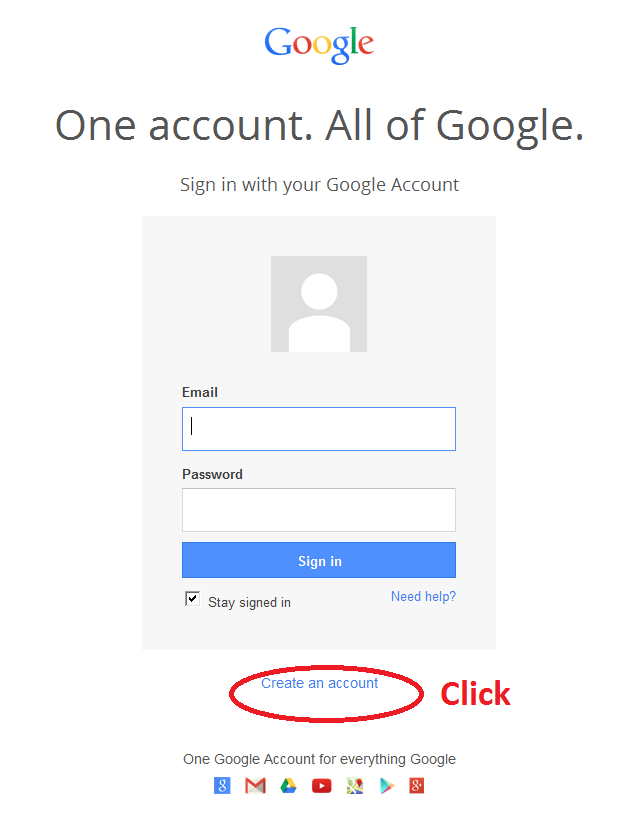The image depicts a Google sign-in dialogue, showcasing distinct components for logging into a Google account. The dialogue features a box labeled "Email or phone" for entering an email address and another labeled "Password" for typing the password. Beneath these input fields, there is a blue rectangular sign-in button with "Sign in" written in white text. Additionally, there's a checkbox labeled "Stay signed in," which can be selected or deselected based on user preference. To the right of the password box, there's a link labeled "Need help?" for users seeking further assistance.

The focal point of the image is a red oval, drawn presumably with a marker, around the "Create account" link, highlighting its importance. Accompanying this oval is the word "click" written in red beside it, directing attention to this option for users who do not yet have a Google account. Below the sign-in options, there's a reminder of various applications accessible once signed in with a Google account, including Gmail, YouTube, and other Google services.